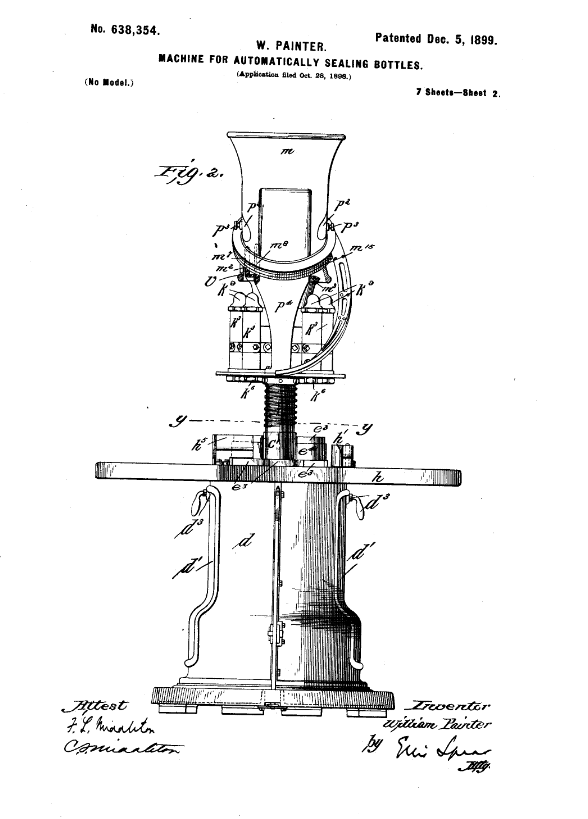The image is a black and white schematic drawing on a white background. Across the top left, it reads "No. 638354," and the top right displays "Patented December 5th, 1899." Centered beneath this, the text "W Painter, machine for automatically sealing bottles" is clearly visible, with unreadable smaller text in parenthesis following it. The left side notes "(No model)" and the right side states "7 sheets, sheet 2." The main drawing features a detailed schematic of a mechanical device designed to automatically seal bottles. The bottle, depicted upside down, appears to be entering a screw-like apparatus. Surrounding the diagram are various notes and indicators, specifying measurements and angles. The structure of the device is quite tall and fairly narrow, with no broad base or platform evident. Along the bottom left, there are indistinguishable signatures, while the bottom right identifies the inventor as "William Painter."